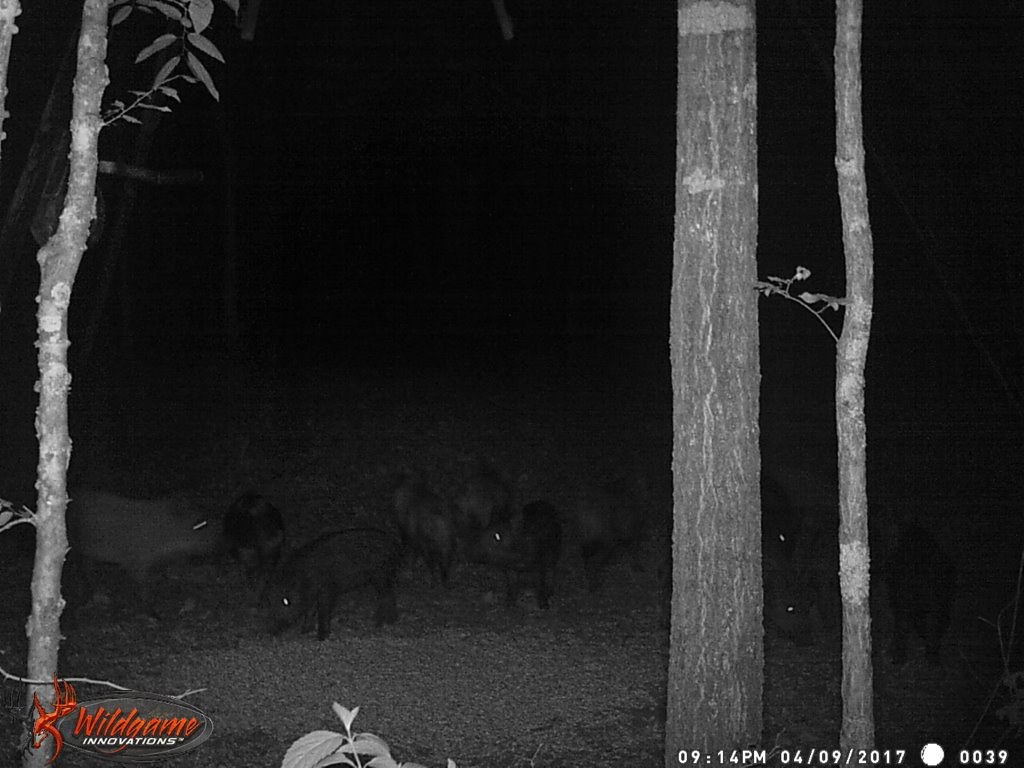The image is a night-time photograph taken with a trail camera, identified as a product from "Wild Game Innovations," whose logo is displayed in the bottom left corner in white and orange. The photograph, dark and mostly in black and white, is time-stamped at 9:14 PM on April 9, 2017, and includes the serial number 0039 in the bottom right. The scene captures a part of a forest with three spindly trees in the immediate foreground, brightly illuminated, along with a small, leafy plant in the lower left corner. In the darker background, approximately 10 wild boars roam, their eyes reflecting the camera's light. The boars appear black, though color details are indistinguishable in the low-light conditions. The image, likely captured to monitor wildlife, emphasizes the wild scene's eerie, nocturnal tranquility, punctuated by the gleaming eyes of the boars and the stark silhouettes of the trees.